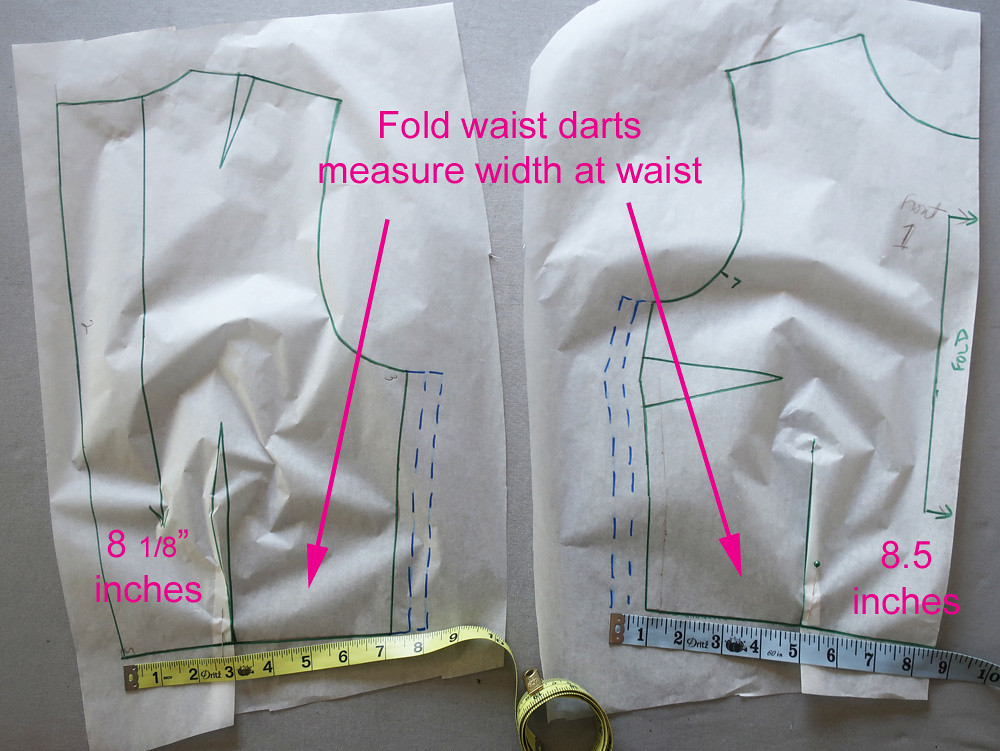The image is a detailed, color photograph of sewing patterns on white tissue paper, designed for a sleeveless vest. The image shows two mirrored patterns for the left and right sides of the vest, each outlined with blue lines and dotted lines. Across the bottom of these patterns are two measuring tapes; a yellow one on the left side measuring 8 and 1/8 inches, and a blue one on the right side measuring 8.5 inches. Pink digital instructions are overlaid on the image, indicating to "fold waist darts" and "measure width at waist" with arrows pointing towards the respective tape measures. Additional notations and markings are present, instructing where to fold and sew the fabric.